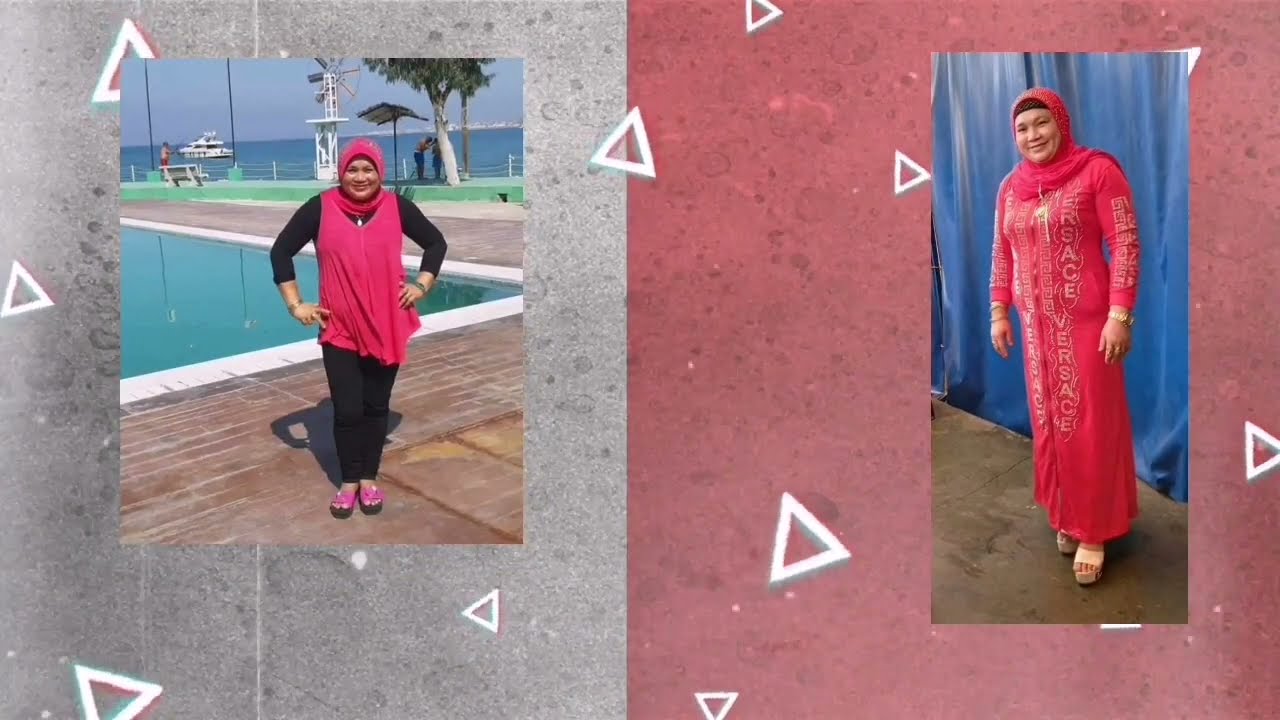The image is divided into two sections with distinct photographs of the same woman, each with unique backgrounds and attire. The left section, bordered by a gray background adorned with white triangles, showcases the woman standing near a swimming pool. Behind her, the scene features an ocean, trees, a windmill, and a ship. She is dressed in a black shirt layered with a red overdress, complemented by a red shawl, black pants, and pink and black slippers. Her head is covered with a pink headscarf.

The right section contrasts with a red background, also marked with white triangles. Here, the woman dons a long, red dress with gold designs and a matching red shawl. A blue cloth hangs in the background, adding to the scene’s vividness. The borders of the photographs enhance the visual separation, with the left bordered in gray and the right in pink. Both photos emphasize the woman's striking attire and varying settings, creating a compelling and detailed comparison.